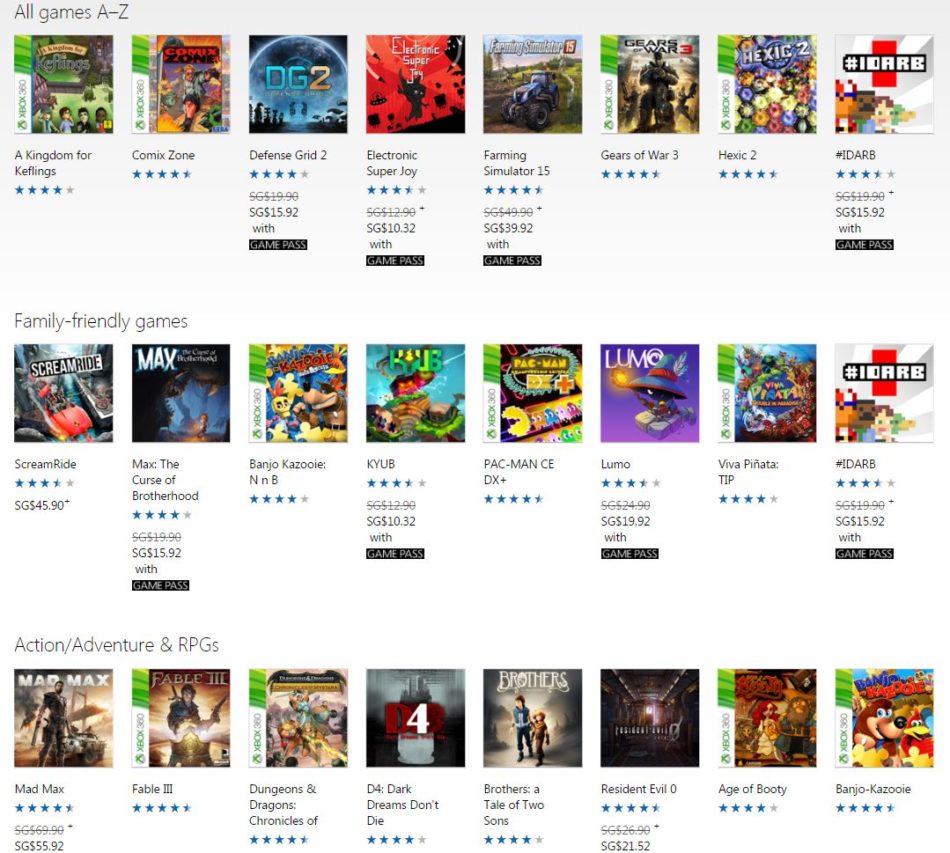A meticulously organized display of video games at a store, showcasing a diverse collection that spans various genres and eras. The selection includes titles such as "Kingdom of Keflings," "Mad Max," "Fable 3," and "Dungeons and Dragons," alongside classics like "Resident Evil Zero" and the whimsically named "Age of Booty," which intriguingly features a gargoyle and a mysterious woman on its cover. Also present is the beloved "Banjo Kazooie," among other lesser-known and seemingly vintage games. This eclectic mix appeals to both seasoned gamers and curious newcomers, hinting at the store's vast and intriguing inventory.